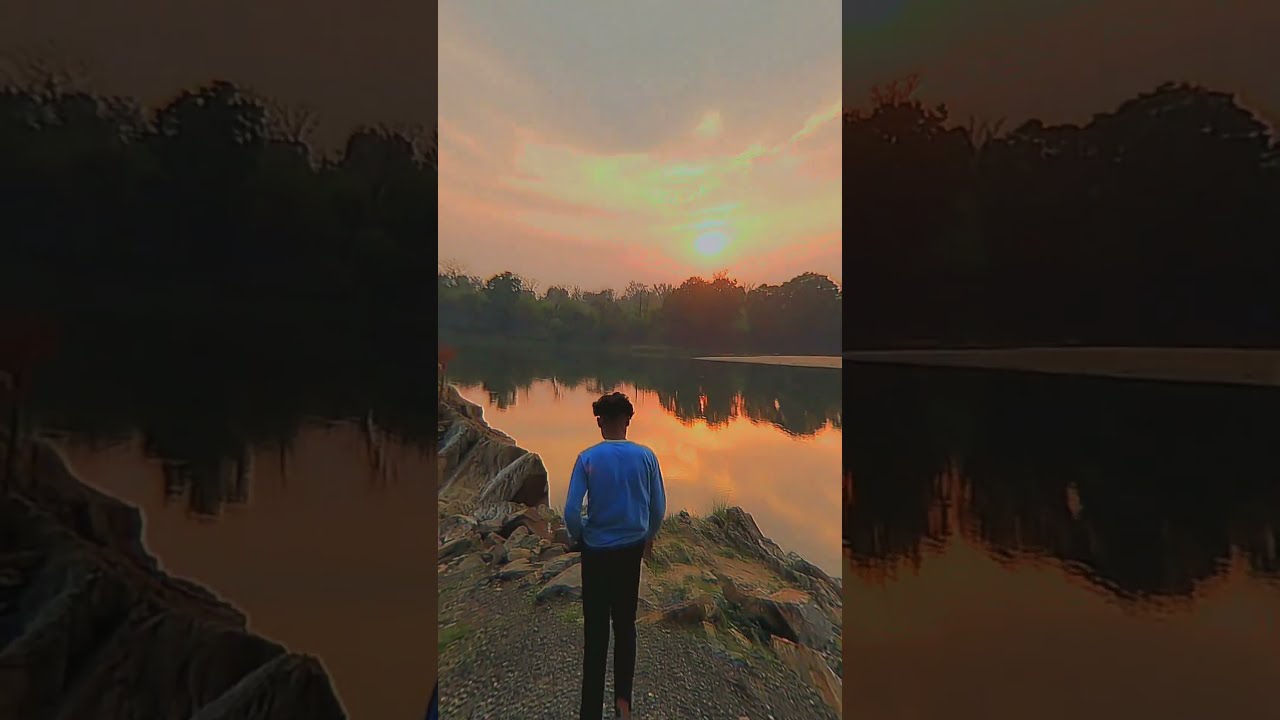The image captures a serene sunset scene by a tranquil lake with the sky painted in shades of orange, yellow, and pink from the setting sun. A young black man, dressed in a blue long-sleeve shirt and black pants, stands on a rocky, jagged shoreline in the center foreground, his back turned towards the camera as he gazes at the picturesque view. The rocks beneath him are a mix of gray, brown, and sandy textures, peppered with tufts of grass. Across the calm water, which perfectly mirrors the radiant colors of the sky and the silhouetted trees lining the opposite shore, the sun peeks just above the treeline, casting a golden glow that enhances the peaceful ambiance of the scene. The gradient sky transitions from warm hues near the horizon to cooler shades with hints of blue, creating a captivating and harmonious composition that evokes a sense of tranquility and wonder.